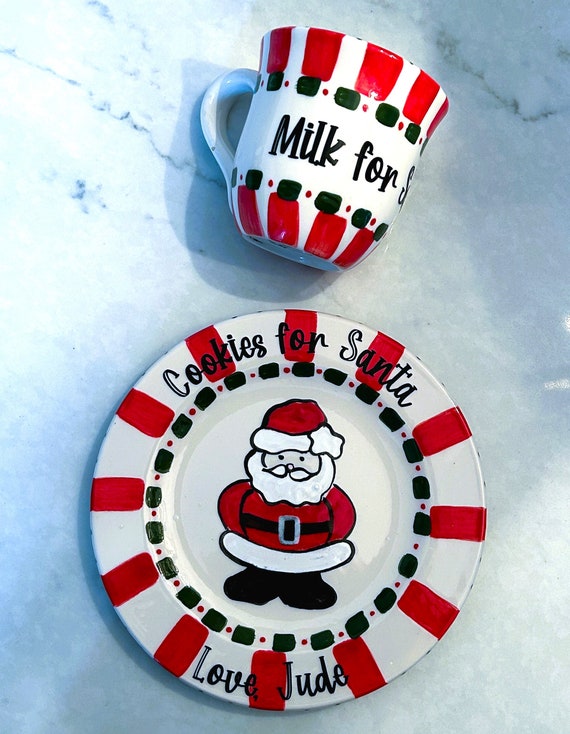The photograph captures an overhead view of a festive setup on a marble countertop, featuring a hand-painted ceramic mug and plate intended for Santa Claus. Both ceramics have a white background with vibrant red and black decorative accents. The mug, which has red vertical stripes at the top and bottom along with horizontal black stripes, is slightly tilted and bears the inscription "Milk for Santa." 

Below the mug, the round white plate also boasts red stripes and black lettering, prominently displaying "Cookies for Santa" at the top and "Love, Jude" at the bottom. In the center of the plate is an endearing, childlike painting of Santa Claus. Santa is depicted in his classic attire with a red hat featuring white fuzzy trim, a matching red jacket with a large buckle and white trim, and black boots. The entire scene exudes a cheerful, Christmassy vibe with its playful artwork and thoughtful messages, all set against the elegant backdrop of the marble countertop.